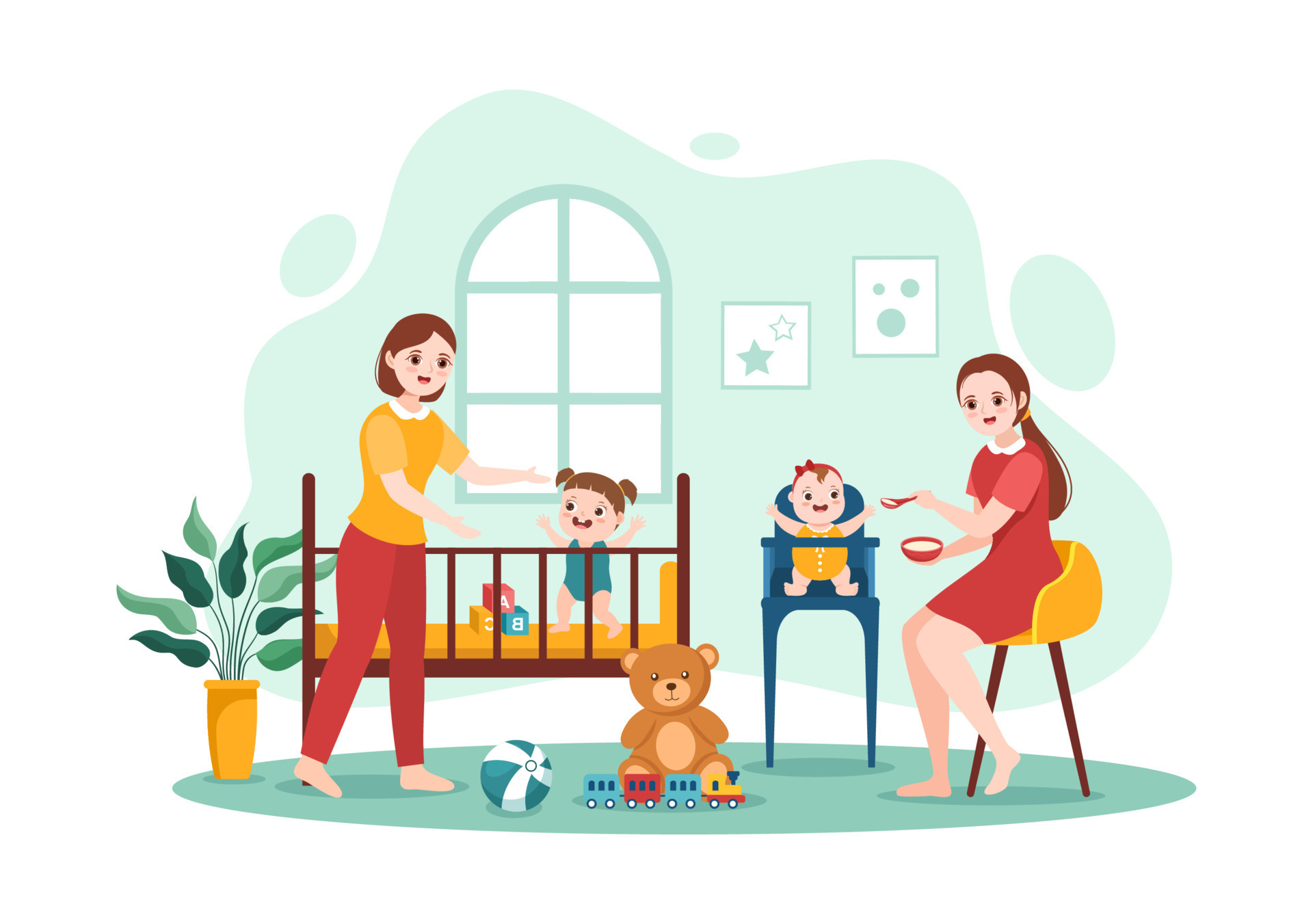In this vibrant, cartoon-style nursery scene, two women are caring for two babies. The background is a mint green with a deeper green rug, creating a cheerful atmosphere enhanced by bright greens, yellows, and rusty reds. The woman sitting on a yellow chair is dressed in a red dress with a white collar and has long brown hair. She is feeding a baby girl in a blue high chair. Meanwhile, another woman, wearing red pants and a yellow shirt, stands barefoot by a crib, engaging with a toddler who is standing and trying to walk towards her. The crib contains three alphabet blocks marked A, B, and C. Scattered on the floor are various toys including a ball, a train set, and a teddy bear that faces the camera. A planter with dark and light green leaves sits at the far left, adding a touch of nature. The room is adorned with a window and two pictures on the wall, completing this cozy and lively nursery illustration.